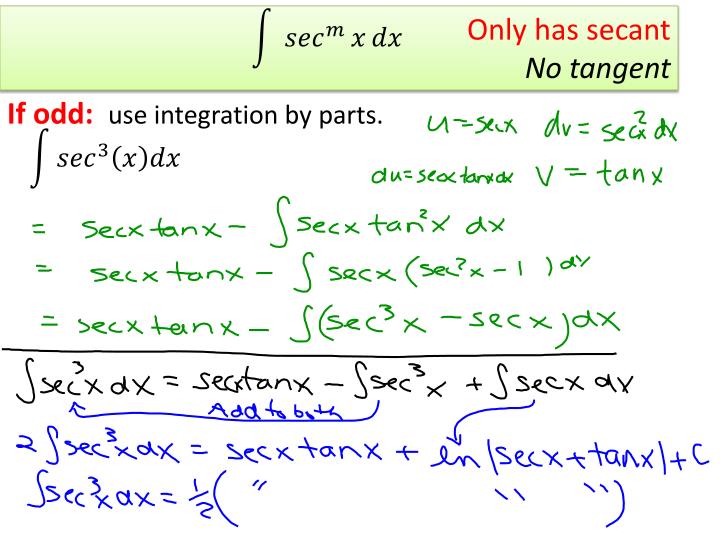This image is a detailed educational infographic in landscape orientation, predominantly focused on trigonometry and integration techniques. At the top, there is a horizontal band with a light green gradient, featuring a centered mathematical notation: "SEC^m(x) dx." In the top right of this band, there is red text stating, "only has secant," while underneath in italicized black text, it reads, "no tangent." Below this, there is a red text annotation that says, "if odd: use integration by parts," followed by the formula, "sec^3(x) dx." The main part of the infographic is filled with a series of handwritten notations and formulas arranged sequentially in green, black, and blue text. The green section includes detailed explanations and calculations, followed by a black handwritten formula and two lines of blue handwritten notations featuring scientific punctuation, equal marks, and fractions. This line art typography infographic provides a comprehensive visual guide to specific trigonometric integration processes, highlighted by its methodical color-coded sections.